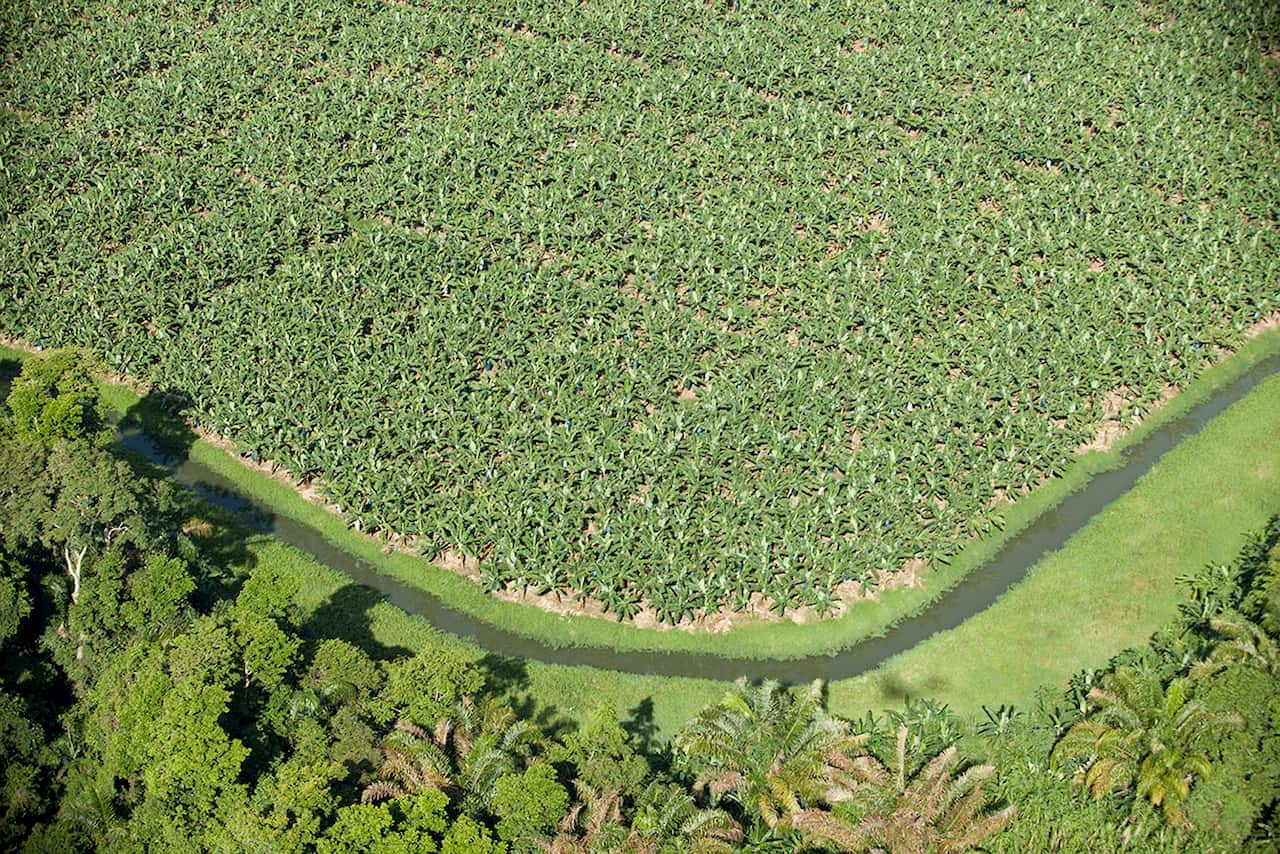The image depicts an aerial view of a well-maintained crop field, likely intended for commercial growth, possibly hemp or another green crop. The field consists of finely trimmed, short plants organized into large, roughly marked rectangles with various lines running through it, suggesting rows or irrigation channels. Surrounding this green expanse is a dark, flowing element that could either be a river, irrigation ditch, or path, giving the appearance of a black walkway. Bordering this outer edge is a dense stand of tall, green leafy trees interspersed with some dry leaves and potential palm fronds or large ferns, casting scattered shadows. The entire scene is bathed in sunlight, illuminating the various green and brown hues of the vegetation, creating a contrast with the darker water or path.